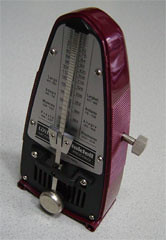The image showcases a vintage metronome in a portrait orientation. The metronome features a dark red casing reminiscent of antique design. Positioned on its right side is a traditional wind-up key, a tell-tale sign of its mechanical nature. The device prominently resembles a classic metronome, with an arch-shaped face and the characteristic pendulum seen in the center. The top section is adorned with a stainless steel plate printed with black numerical markings and scales, indicative of its function to measure tempos. The overall structure shares a likeness to a Brannock device (used for shoe sizing), especially in its shape and arched dial area. The lower segment of the metronome is black, with small vent-like openings. This detailed context suggests a classic, wind-up metronome, potentially without electronic features such as a backup battery or auditory beat announcements.